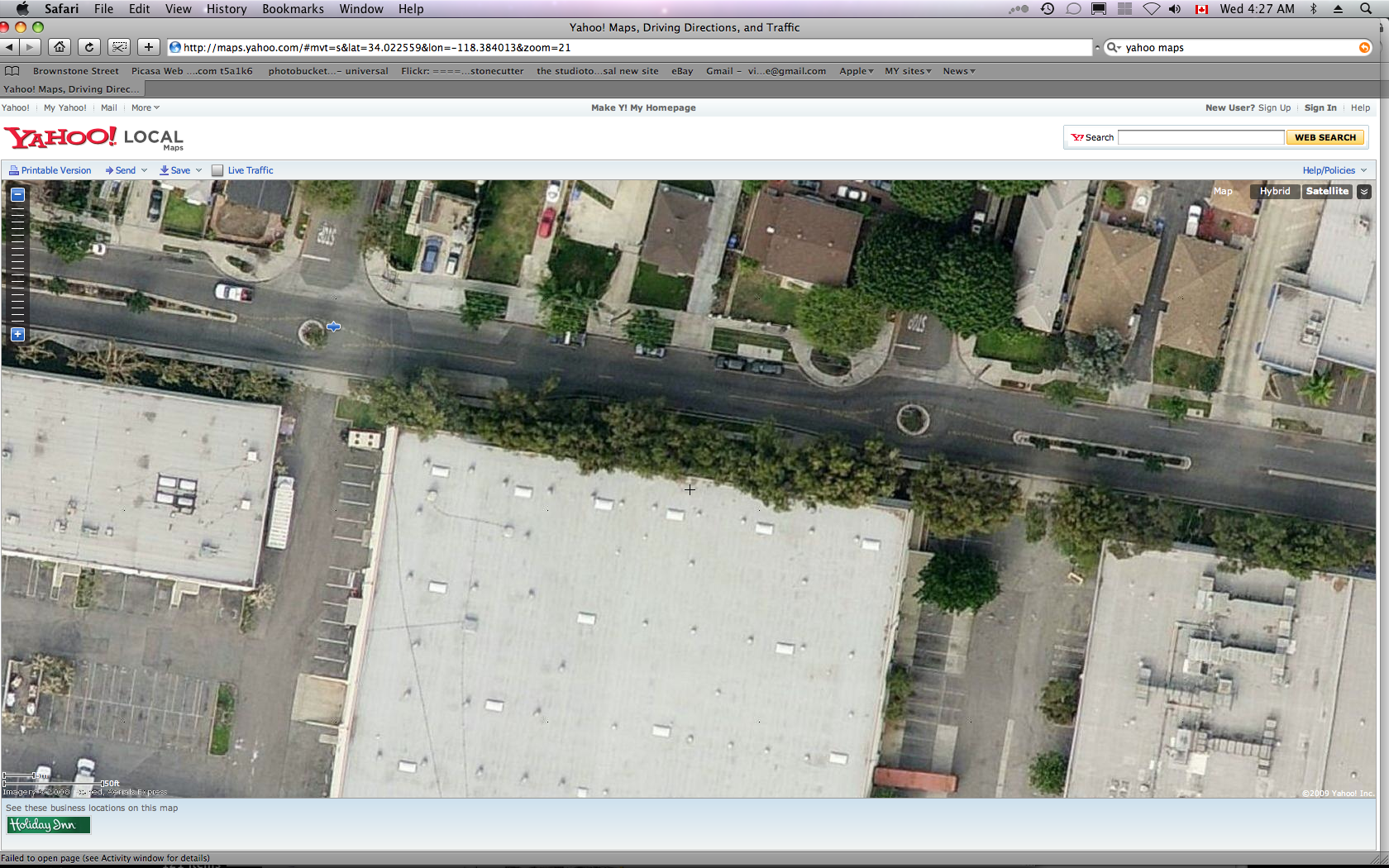An overhead map view displayed on Yahoo Maps in the Safari browser on an Apple computer. The image showcases a mixed landscape of urban and suburban elements divided by a central street running horizontally across the middle. At the bottom of the screen, there are three large commercial buildings with flat rooftops, possibly accessible on foot, accompanied by visible parking spaces. Across the street, which features medians and several moving vehicles, lies a residential neighborhood. This area comprises seven distinct houses with driveways and a few parked cars. Additionally, the top right corner reveals part of another store with a flat roof and adjoining parking spaces. The scene is interspersed with numerous trees lining the road and scattered between the houses, partially obscuring certain sections of the street.